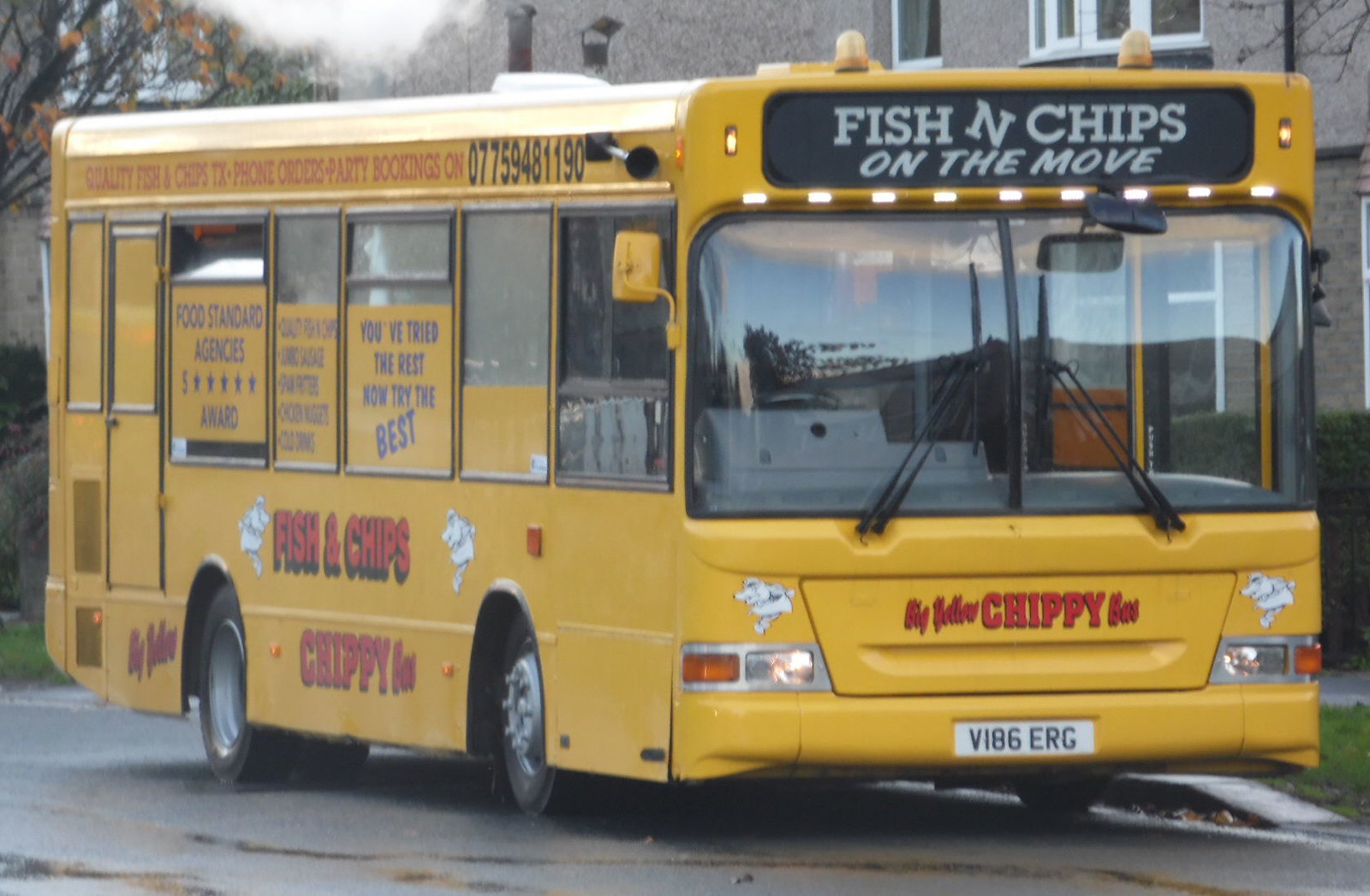This outdoor, daytime image features a repurposed city bus situated centrally on an asphalt road. The bus, now a mobile food truck advertising "Fish and Chips on the Move," dominates the scene. Visible text on the bus includes slogans like "You've tried the rest, now try the best" and "Quality fish and chips in Texas," as well as contact information: 077-594-81190 for phone orders and party bookings. The bus windows also display a Food Standards Agency five-star award. Surrounding the bus, the image reveals patches of grass, a sidewalk, and some bushes leading to a building in the upper right corner. The color palette is a mix of gray, yellow, red, black, white, blue, and orange, reflecting various elements of the bus and its advertisements. The scene suggests the bus is in the UK, inferred from the license plate, despite the Texas reference.